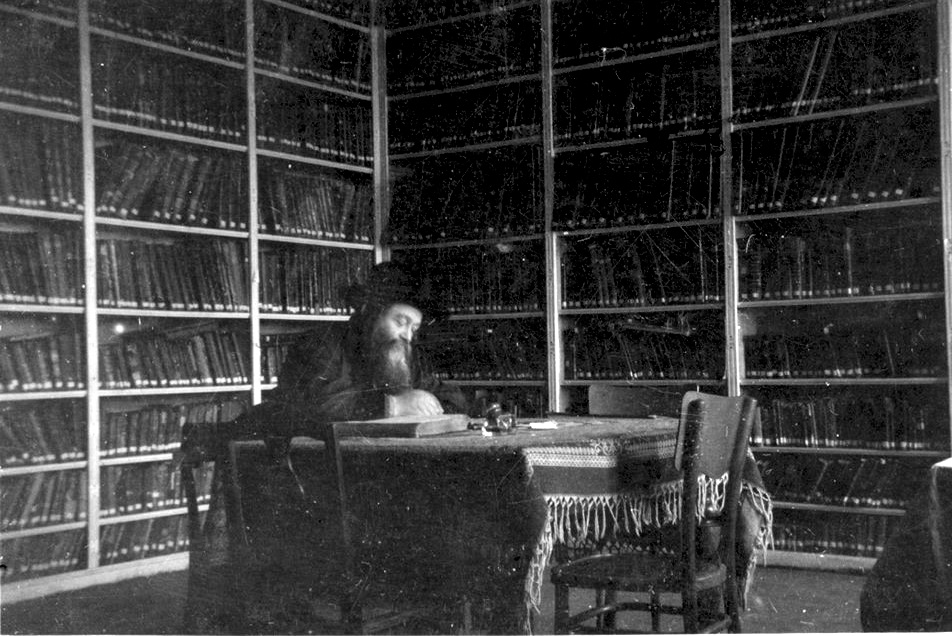The black and white photo captures a solitary Jewish man, possibly a rabbi, deeply engrossed in studying a scripture. Seated on one of the chairs that surround a table covered with a fringed tablecloth, he reads from an open book. The man, with a long beard graying at the ends, sits at a table positioned at the meeting corner of two large bookshelves that dominate the background. These bookshelves, standing at least seven to eight shelves high, are filled with books from top to bottom. The overall clarity of the image is remarkable, with ample lighting accentuating the serene and studious atmosphere of the room.